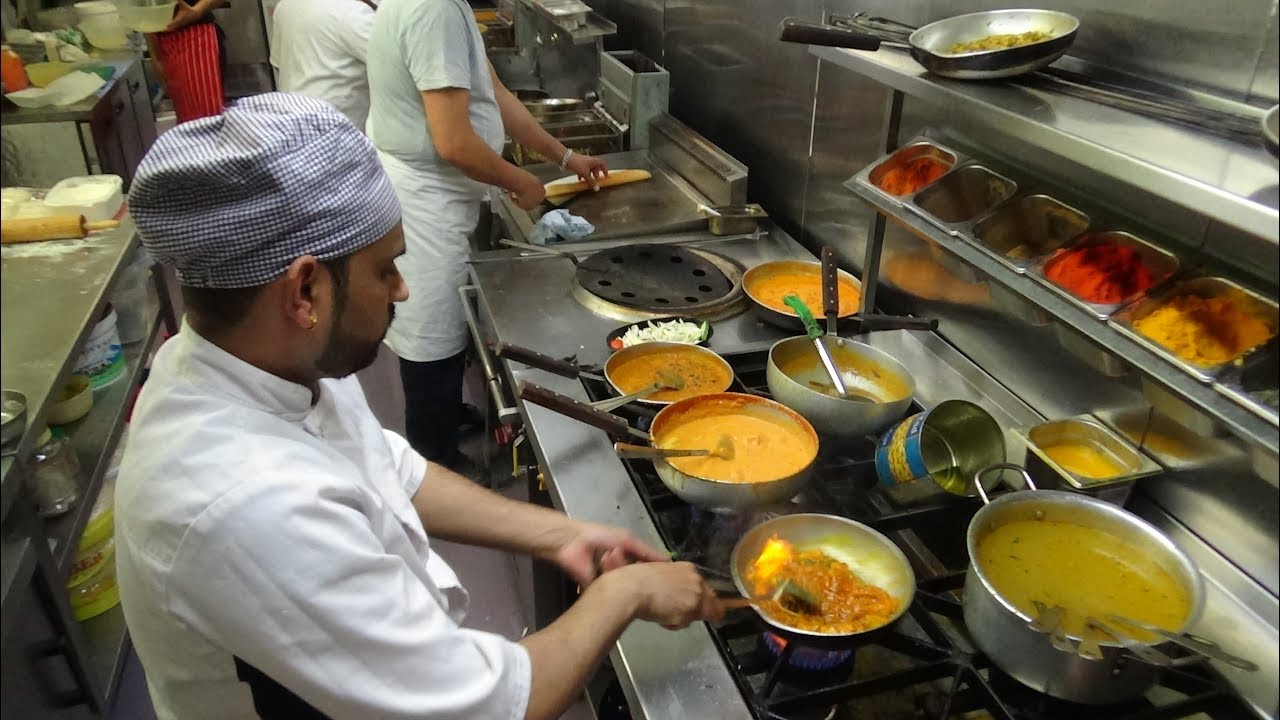This image captures a bustling kitchen scene in what appears to be an upscale restaurant. Three chefs are actively engaged in various culinary tasks. In the foreground, a chef with a blue and white checkered cap and a white shirt is stirring a brown sauce in a saucepan on the stove. Surrounding him are multiple pots and pans containing various dishes, including a tomato-based sauce, a green soup, an orange sauce, and a pot that looks like chicken broth. He has a medium olive-brown complexion, a beard, and appears to be focused on his task.

Behind him, the bodies of two other chefs are visible, though their heads are cut off in the image. Both are clad in white shirts, aprons, and black pants. One appears to be slicing a baguette, while the activity of the other remains unclear. The kitchen is well-equipped with silver industrial equipment, including a rolling pin and a container of flour. Alongside the wall, there are trays containing assorted vegetables such as green, yellow, and red bell peppers, cucumbers, and other items. A shelving unit stacked with different-sized containers can also be seen in the background, contributing to the organized yet busy atmosphere of this upscale kitchen.